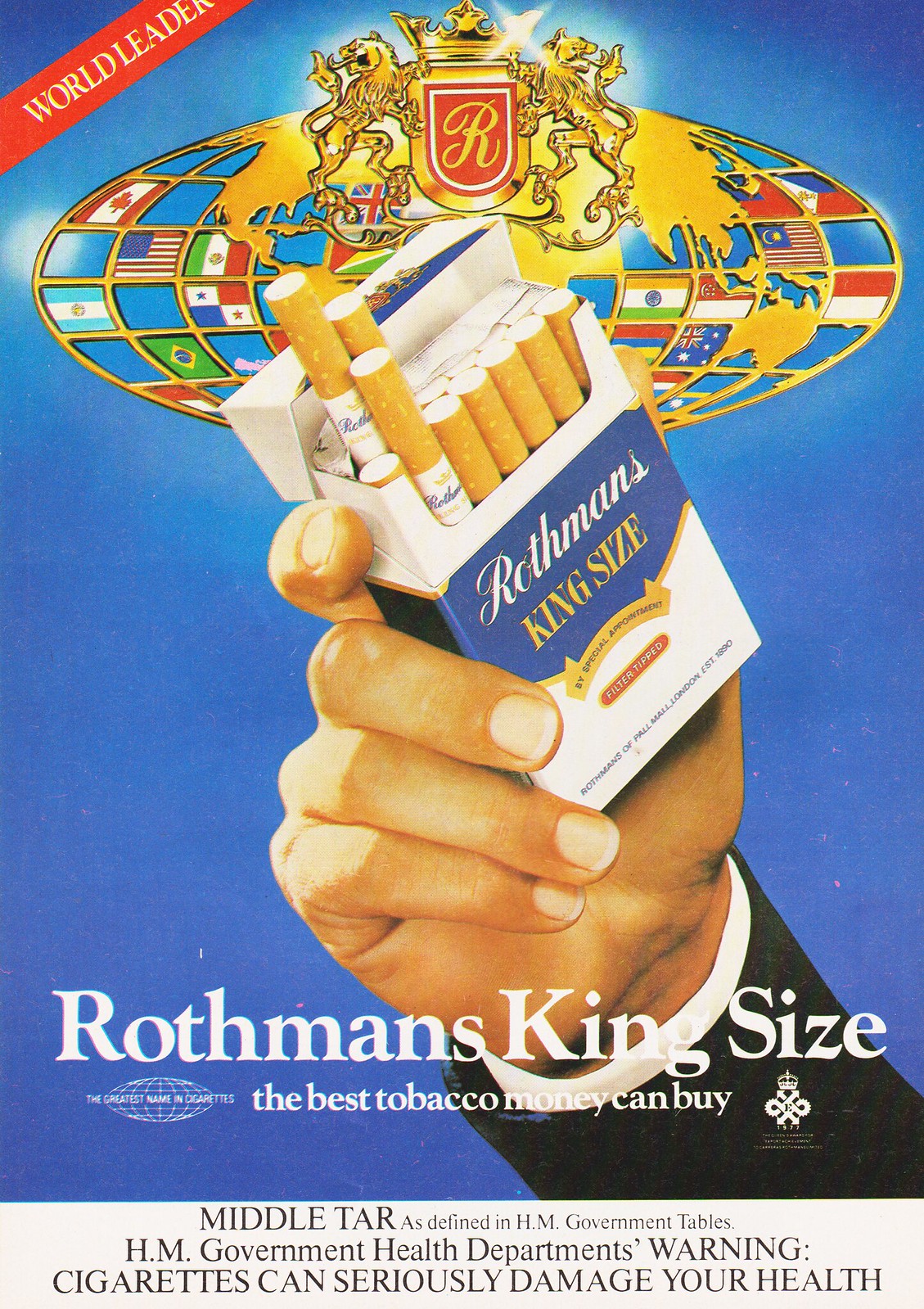The image appears to be a scan of an advertisement from an old magazine, featuring a colorful, well-preserved yet slightly scratched design. At the center is an open carton of Rothman's King Size cigarettes, with three cigarettes partially pulled out, showing white bodies and brown filters. The carton, predominantly white with blue trim, is held by a hand clad in a black suit with a white undershirt and cufflinks, suggesting the hand belongs to a businessman.

In the background, there's a globe depicted in gold with numerous country flags adorning it. Above the globe is a red shield adorned with a gold 'R' and crowned, flanked by two gold lions with their tongues out. At the top left corner of the advertisement, the text reads "World Leader" in white. The Rothman’s logo is prominently displayed above the globe.

At the bottom of the advertisement, in white text against a contrasting background, it states, "Rothman's King size. The best tobacco money can buy. The greatest name in cigarettes." Below this, in black text, it continues, "Middle tar as defined in HM government tables. HM government health department's warning: Cigarettes can seriously damage your health."

The overall impression suggests a nostalgic yet sophisticated promotional piece, emphasizing both the luxury and the health risks associated with smoking.